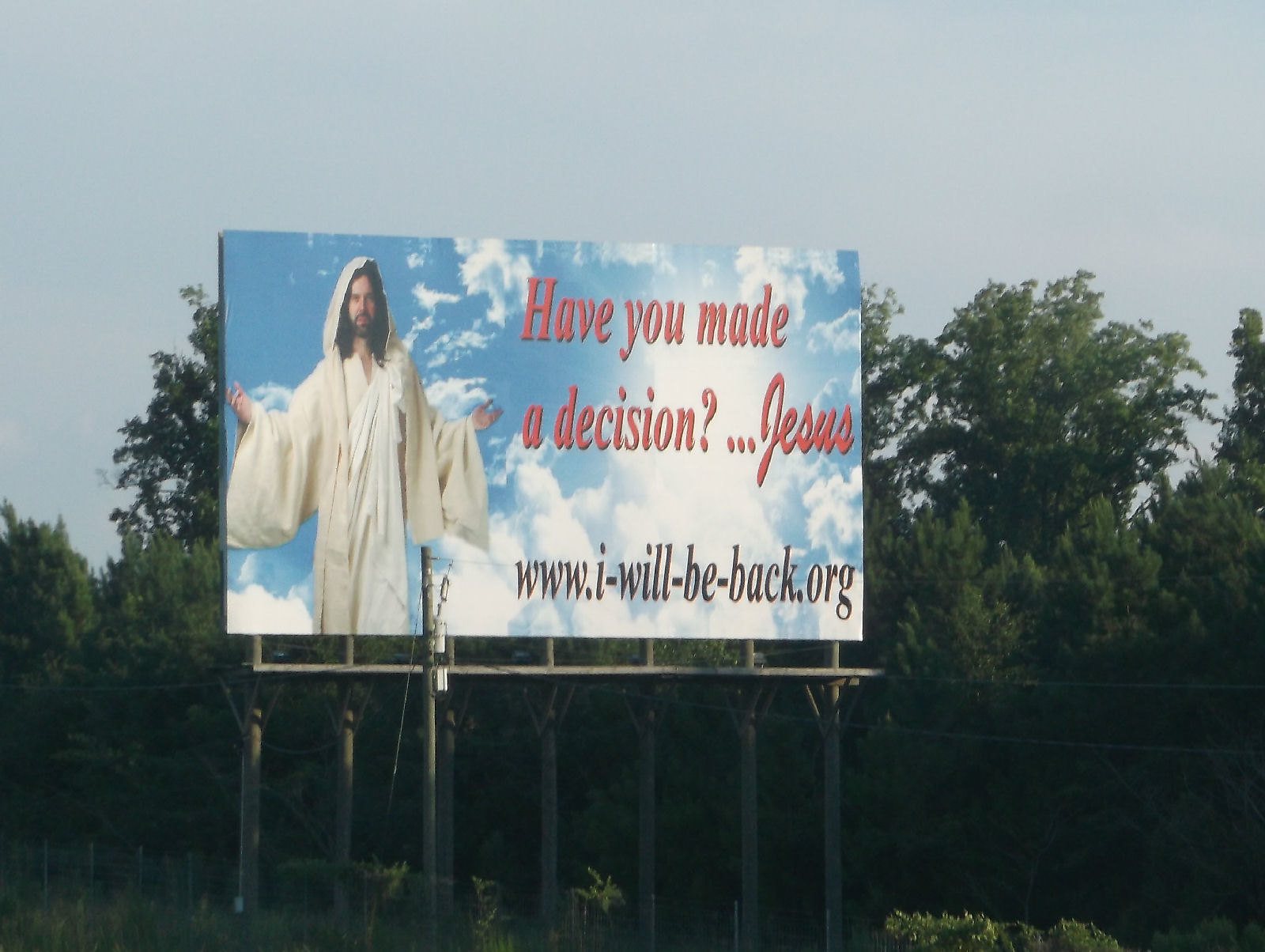This image captures a large rectangular billboard situated along a highway. The billboard prominently features a depiction of a man dressed as Jesus, a white Caucasian male, wearing a white robe with his arms raised. The backdrop of the billboard shows a somewhat murky blue sky with sparse clouds. In bold red font, the text reads: "Have you made a decision? ... Jesus." Below this text, the web address "www.i-will-b-back.org" is displayed. The billboard is supported by a wooden frame comprised of seven individual dark brown wooden legs. In the background, you can see a scenic view with trees, telephone poles, and various types of vegetation, all contributing to the rustic atmosphere surrounding the billboard. The overall tone of the sky hints at a day that is neither particularly bright nor overcast.